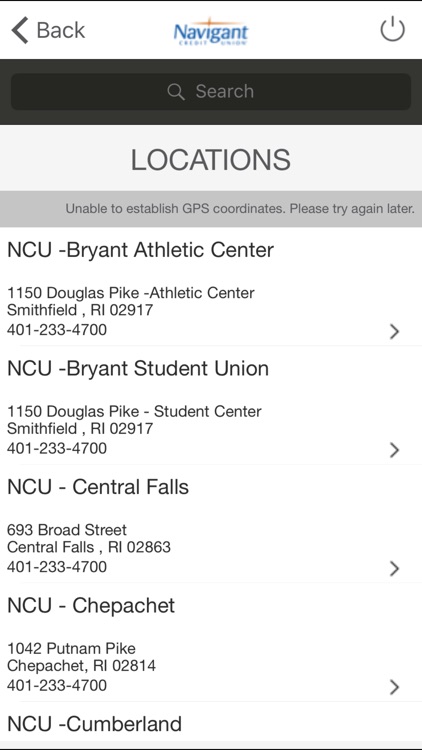This screenshot displays the interface of the Navigant app, identifiable by the distinctive blue Navigant logo positioned in the upper middle section of the screen. The app navigation bar is evident at the top, featuring a "Back" button with a left-pointing arrow on the left and a power toggle on the right. Directly below is a prominent black search bar.

The header "LOCATIONS" is clearly marked in dark gray uppercase letters beneath the search bar. Below it, a notification indicates, "Unable to establish GPS coordinates, please try again later." Listed thereafter are several locations, each with detailed information:

1. **NCU Bryant Athletic Center**
    - **Address:** 1150 Douglas Pike Athletic Center, Smithfield, Rhode Island, 02917
    - **Phone Number:** 401-233-4700
    - **Navigation:** A right-pointing arrow suggests more details can be accessed.
   
2. **NCU Bryant Student Union**
    - **Address:** Provided
    - **Phone Number:** Provided
    - **Navigation:** Right-pointing arrow for more information.
   
3. **NCU Central Falls**
    - **Address:** Provided
    - **Phone Number:** Provided
    - **Navigation:** Right-pointing arrow for more information.
    
4. **NCU Cheepachet**
    - **Address:** Provided
    - **Phone Number:** Provided
    - **Navigation:** Right-pointing arrow for more information.
    
The last entry, **NCU Cumberland**, is truncated, leaving the contact information incomplete and not visible.

This comprehensive layout allows users to easily identify and access various Navigant Credit Union locations along with their respective addresses and phone numbers.